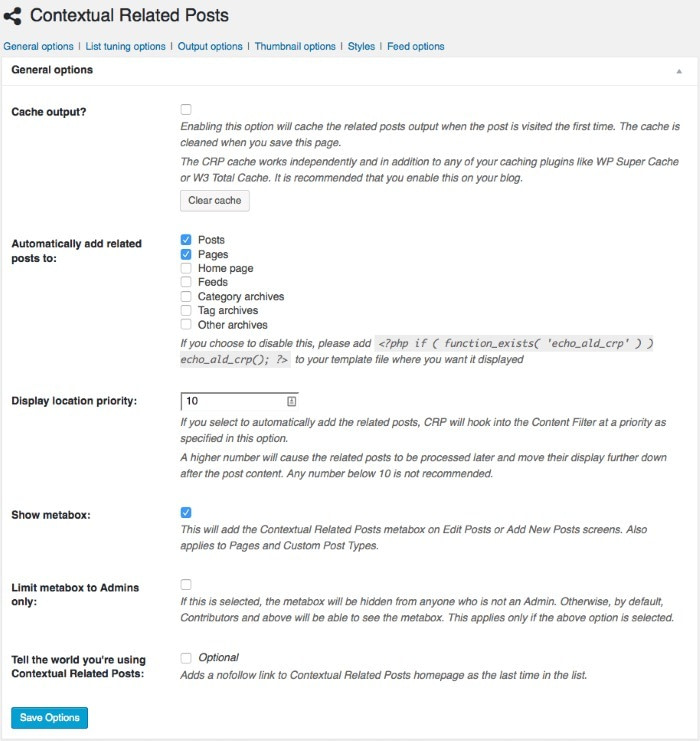The image captures a computer screen displaying the "Contextual Related Posts" settings page on a website. The user is currently within the "General Options" tab. On the left side, there are various black headings indicating different sections of settings. To the right of these headings, the interface allows users to make detailed selections pertaining to the functionality of contextual related posts. 

At the very bottom of this interface, there is a prominent blue button labeled "Save Options." The specific settings available on this page include:

1. **Cache Output**: Offers an option to clear the cache and a checkbox enabling the caching of related posts when the post is visited for the first time.
2. **Automatically Add Related Posts To**: This section features multiple items to check, with "Posts" and "Pages" currently selected by default via blue checkmarks. Additional selectable options include "Homepage" and "Feeds."
3. **Display Location Priority**: Contains an input field where users can designate a priority number.
4. **Show Meta Box**: A checkbox option to display a meta box.
5. **Limit Meta Box to Admins Only**: This option is displayed but presently not selected.
6. **Tell the World You're Using Contextual Related Posts**: An unselected checkbox option allowing users to publicly share that they are utilizing this feature.

This detailed settings interface enables users to fine-tune their related posts' functionality and display, ensuring a tailored content-sharing experience.